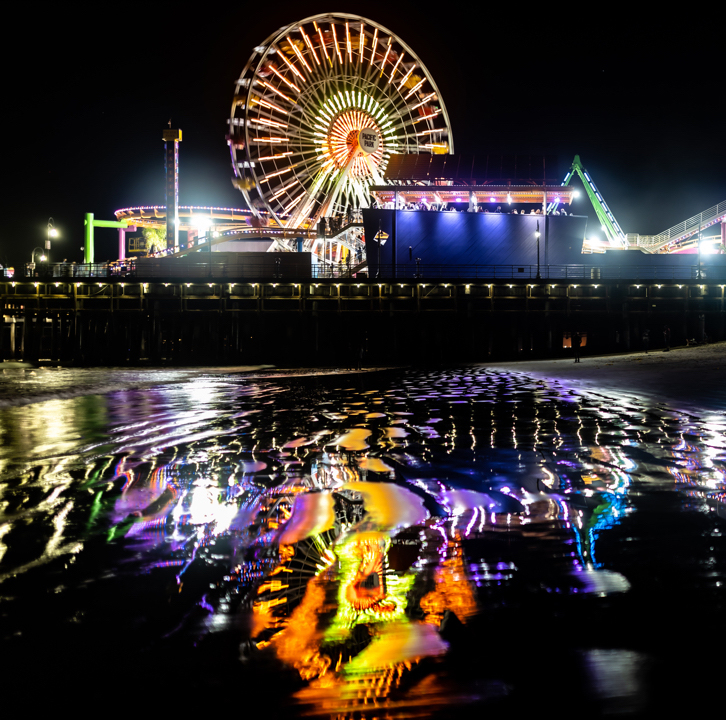The image captures a vibrant carnival scene set atop a pier extending over a beach, likely reminiscent of locations in California. Dominating the foreground is a large, illuminated Ferris wheel with red and yellow seat cars. The Ferris wheel’s bright, colorful lights cast vivid reflections of orange, yellow, purple, and blue onto the rippling water below. To the right of the Ferris wheel, a green roller coaster's track twists and peaks against the night sky, highlighting a thrilling descent towards a brightly-lit booth. Additional attractions include a multicolored carousel with a prominent orange center and a yellow outer ring, as well as another ride with long, green, extended arms. Neon-lit buildings below the carousel add a further splash of orange, contributing to the lively reflections in the water. The overall ambiance is one of dazzling lights and dynamic colors, all set against the dark, nocturnal backdrop of the ocean.